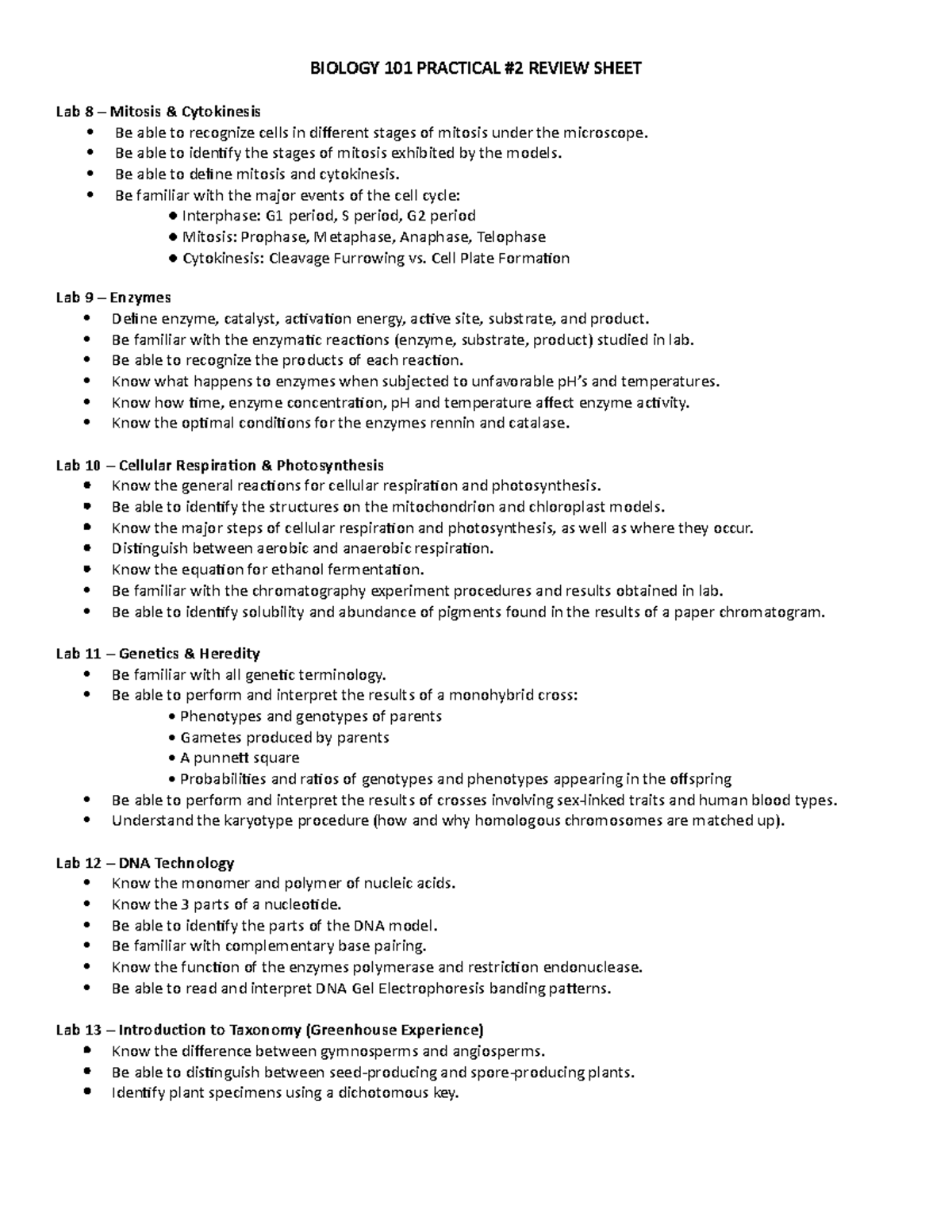A detailed, cleaned-up caption for this image could be:

---

The image depicts a full-page school form titled "Biology 101 Practical, Number 2 Review Sheet" against a plain white background. The text is extremely small, making it somewhat difficult to decipher. The first heading, which is bold and prominently highlighted, reads "Lab 8: Mitosis and Cytokinesis." Below this heading, there are four main bullet points. The fourth main bullet point further breaks down into three additional sub-points. The subsequent section is labeled "Lab 9: Enzymes," featuring approximately six to eight bulleted sentences. Following this, "Lab 10: Cellular Respiration and Photosynthesis" is outlined, including another set of around eight highlighted sections. The review sheet continues with "Lab 11: Genetics and Heredity," followed by "Lab 12: DNA Technology." Finally, "Lab 13: Introduction to Greenhouse Experience" is mentioned. The entire page is densely packed with information, structured to guide students through various key topics covered in the Biology 101 practical course.